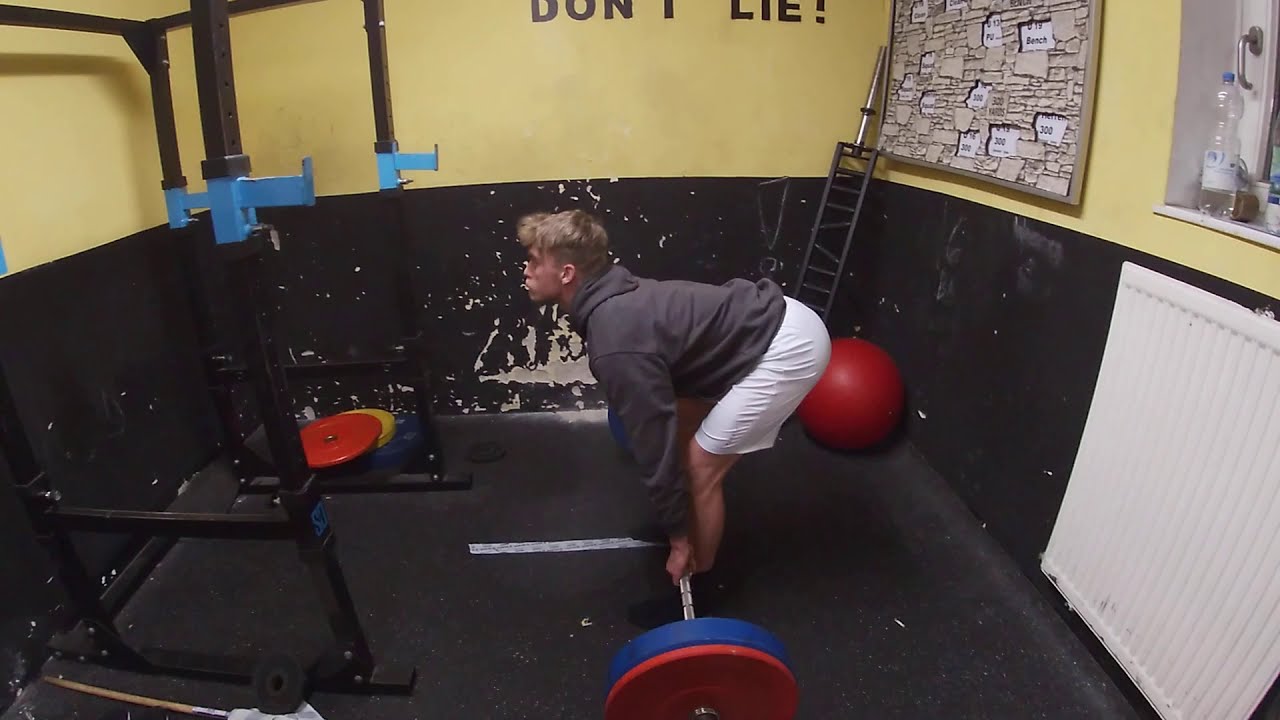A young man, dressed in a grey long-sleeved hoodie with the hood down and white shorts, is positioned to lift a heavy silver chrome barbell with blue and red circular weights on each end. He is bent over with a level back and his rear end sticking out to the right. The setting is a weight room with a black floor. In the background, the room features yellow walls on the top and black walls on the bottom, the latter of which is peeling and scuffed. Behind him to the right, a red exercise ball sits in the corner next to a rectangular metal structure with a silver bar at the top. A white vent is visible on the lower right side of the wall, and an indented shelf holds an empty water bottle above which a silver handle is mounted. Adjacent to it is a corkboard with patches and numbers, including the number 300 in black text. In the center of the wall, the phrase "Don't lie!" is boldly displayed in black text. To the left, a metal rack with blue hooks three-quarters up holds additional weights, including a red and a yellow dumbbell in the upper left corner.